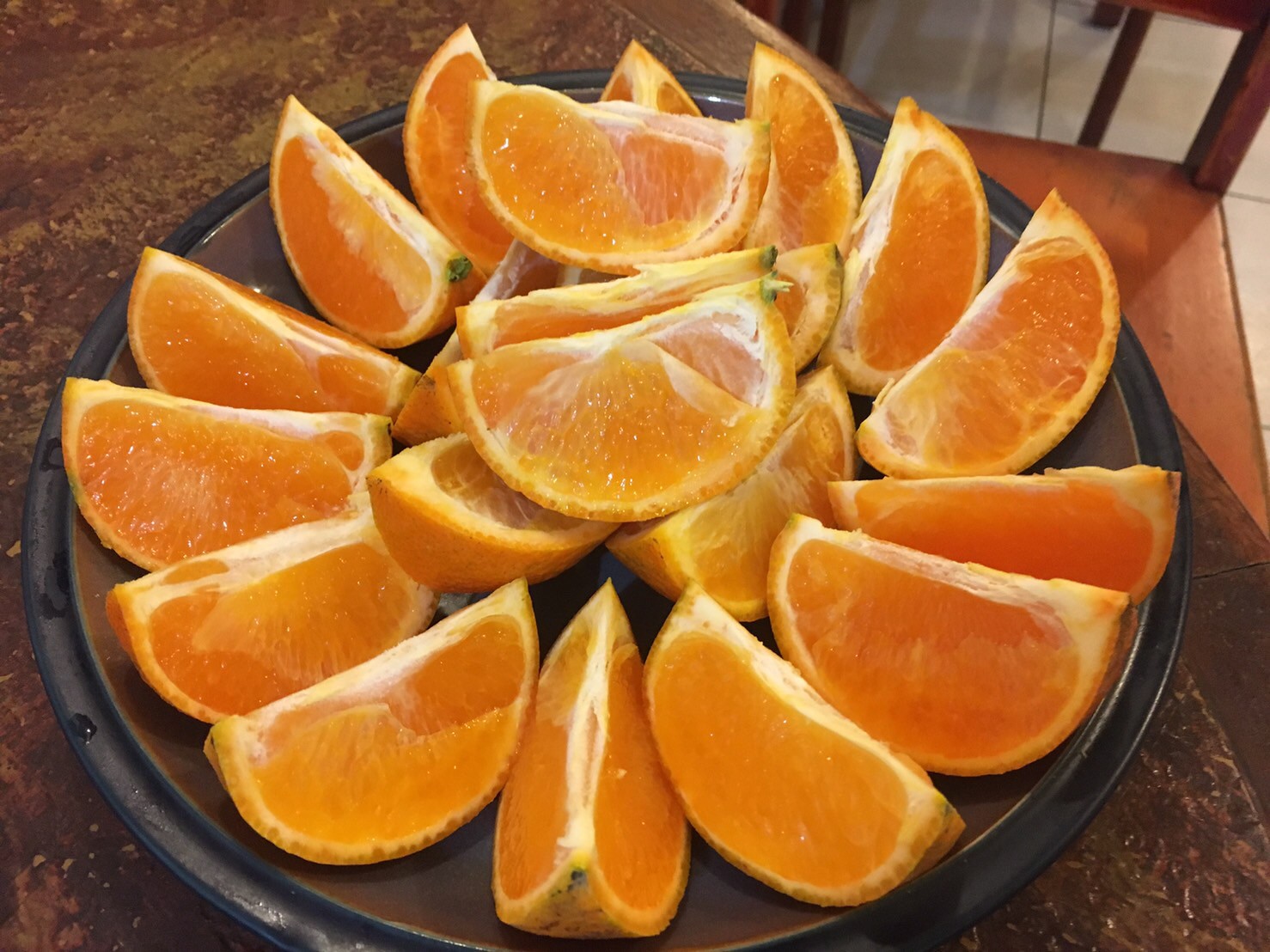This image presents a neatly arranged display of approximately 15 orange slices on a dark, possibly black or very dark brown, plate that rests on what appears to be a wooden table. The slices, likely from two large oranges, are meticulously arranged in a circular pattern around the outer edge of the plate, with additional slices stacked in the center. The table itself is a rich, wooden brown, enhancing the warm tones of the orange slices. In the background, notably in the top right-hand corner, a section of a wooden chair is visible. The floor beneath is light-colored, either white or pale tiles, providing a subtle contrast against the wooden elements of the scene.